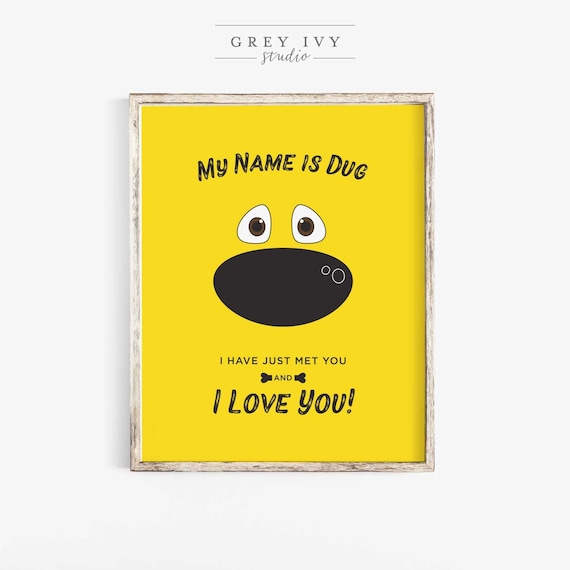This photograph captures a vibrant mustard yellow poster framed in a weathered white wood frame, created by Gray Ivy Studio. The text on the poster, printed in black, introduces a character named Doug with the words: "My name is Doug. I have just met you, and I love you." The artwork features an illustration resembling a dog's face, with pupils accentuated by their white scleras, providing the only contrast on the otherwise monochromatic text and image. The scene is further anchored by the inscription "Gray Ivy Studio" at the top of the frame, lending a textured and cohesive artistic feel to the composition.